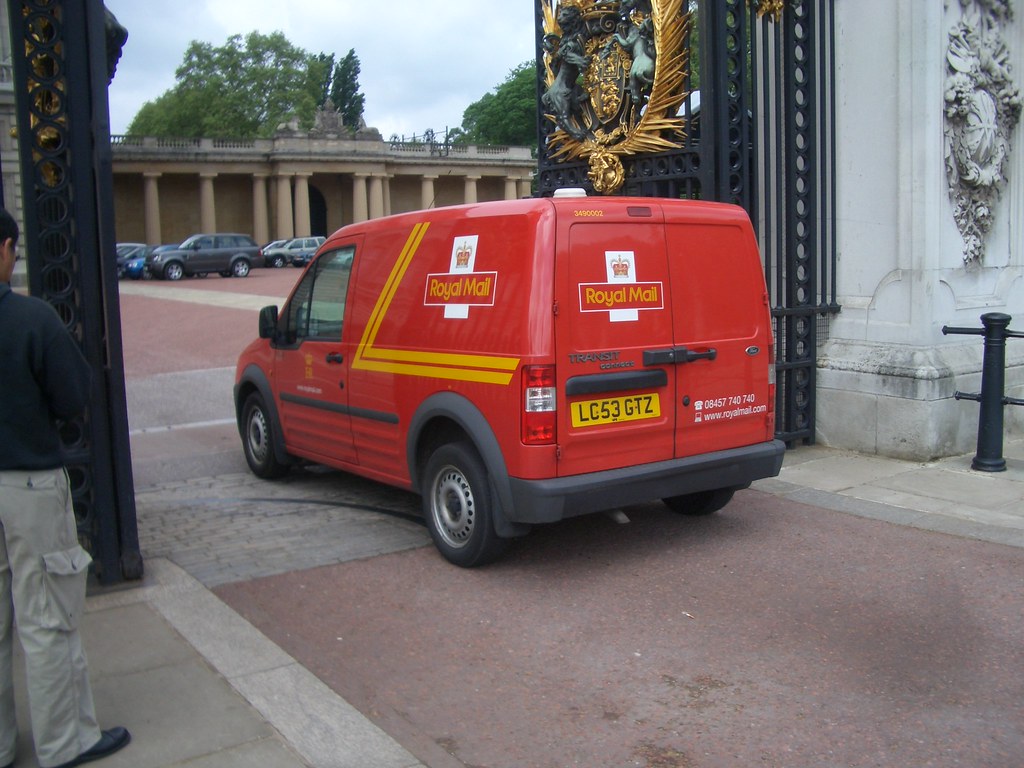The photograph captures a vibrant scene set outdoors, featuring a distinctive red Royal Mail postal van adorned with yellow striping and the Royal Mail logo with an English crown. The van is passing through an imposing ornamental black iron gate that stands approximately 20 feet high, intricately decorated with golden heraldry including crowns, shields, and lions, suggesting a connection to British royalty. To the left of the frame, there is a partially visible man dressed in grey cargo pants and a black sweater. Beyond the grand gates, a courtyard filled with parked cars can be seen, surrounded by thick, decorated pillars, hinting at a possibly governmental or royal property. The scene reflects a meticulous blend of opulence and everyday duty, with the Royal Mail van dutifully carrying out its deliveries within a regal environment.